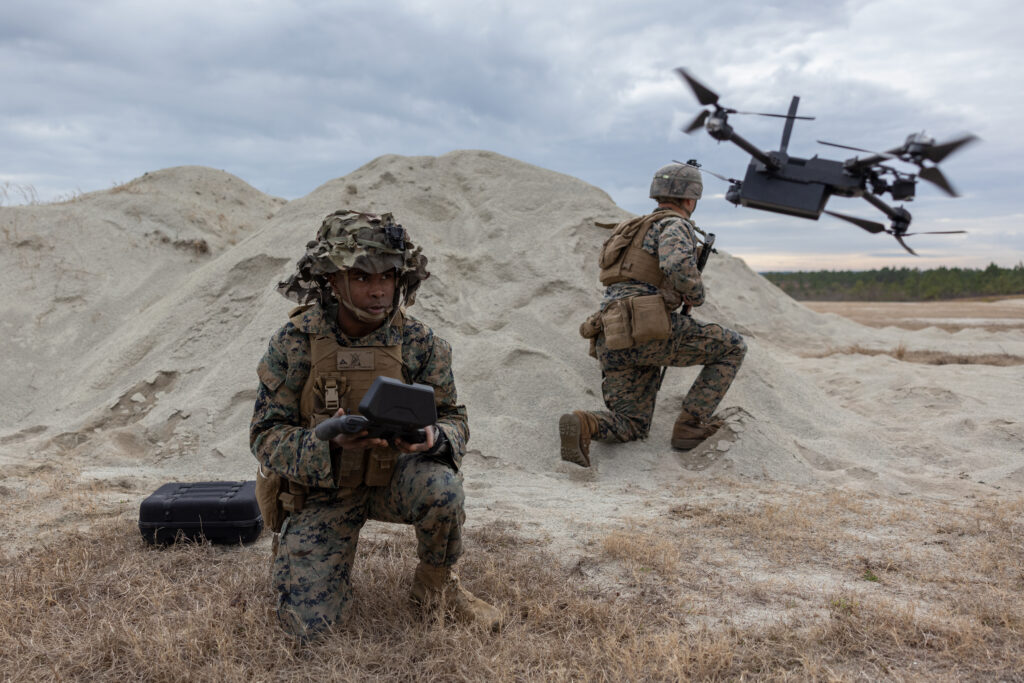The photograph captures a detailed scene of two soldiers crouched behind a mound of tannish-white sand in what appears to be a desert environment, possibly during a military exercise or mission. Both soldiers are clad in full military uniforms with sand camouflage patterns. The soldier in the foreground, kneeling and facing the camera, is holding a black electronic controller, seemingly maneuvering a black drone or special military helicopter hovering low in the sky above them. He sports a wide-brimmed, camouflaged hat and has a black suitcase next to him. In contrast, the soldier positioned behind him is also kneeling, but facing outward, monitoring the situation with a combat helmet, tan vest, and additional gear attached to his belt. The scene features a daytime sky with plenty of clouds, and the background reveals patches of green foliage, hinting at a semi-arid terrain.